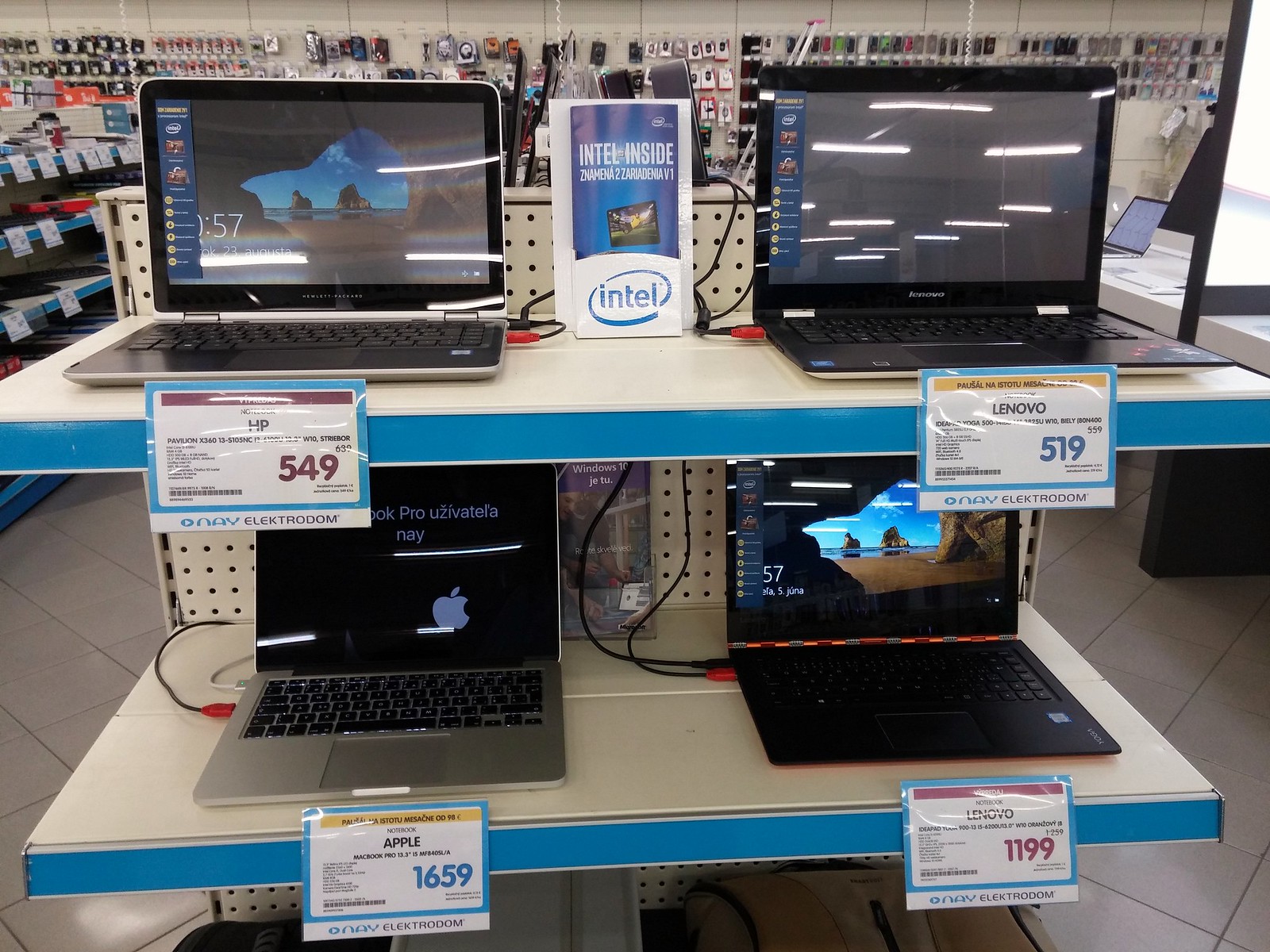This image depicts an electronics store, focusing on a three-shelf end cap display featuring four laptops. The store's floor is tiled, and the shelving is white with blue accents and metal pegboard backing. The top shelf houses an HP Pavilion x360 priced at $549 on the left with its screen showing a beach picture, and a Lenovo Ideapad Yoga 500 priced at $519 on the right, which is turned off, reflecting the store’s fluorescent lights. Between them, an Intel brochure bearing "Intel Inside" is visible. The middle shelf displays an Apple MacBook Pro on the left, showcasing a partially obscured screen with "MacBook Pro" in a foreign language and priced at $1,659. To its right, a Lenovo laptop, also turned on, bears a sticker and is priced at $1,199. The bottom shelf is mostly cut off, but pricing labels suggest more products. The backdrop reveals various electronic accessories such as phone covers, chargers, and possibly printers, organized on hooks along the back wall. The aisles on either side of the display hint at additional products and signage.